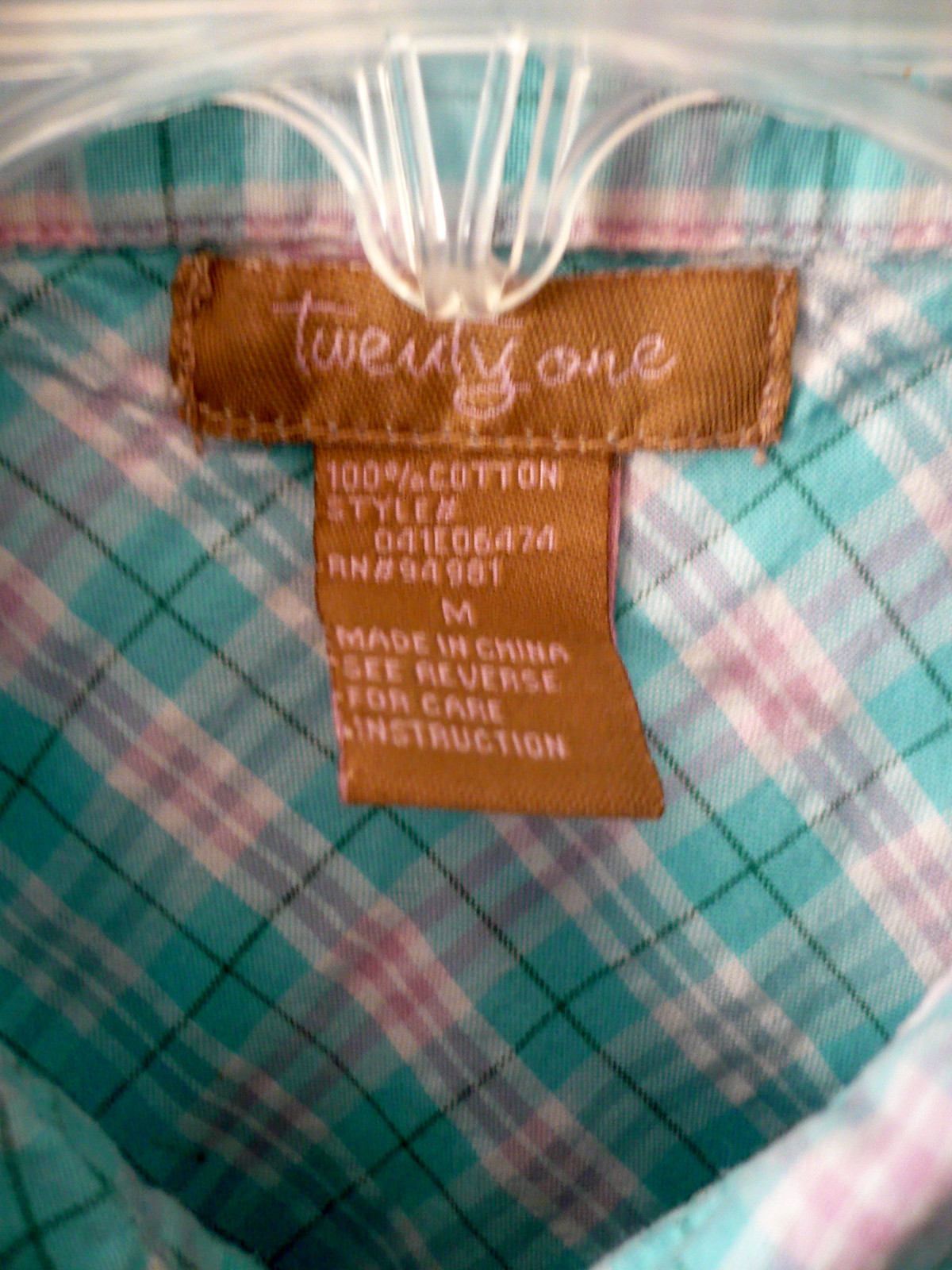The photo features a vibrant, diagonally plaid garment hanging from a handle. The plaid pattern incorporates a mix of turquoise, pink, white, and black lines. The garment is attached to a plastic hanger, the top portion of which is partially cut off in the image. Prominently displayed on the garment is an orange label bearing the text “White Script 21.” Below this label, there's a smaller, similarly colored label that indicates the garment is “100% cotton” and includes style details along with serial numbers. The label also specifies that the garment is a medium size, made in China, and advises to see the reverse side for care instructions. The garment’s corners are slightly rounded, although the exact type of garment remains unclear from the image alone.